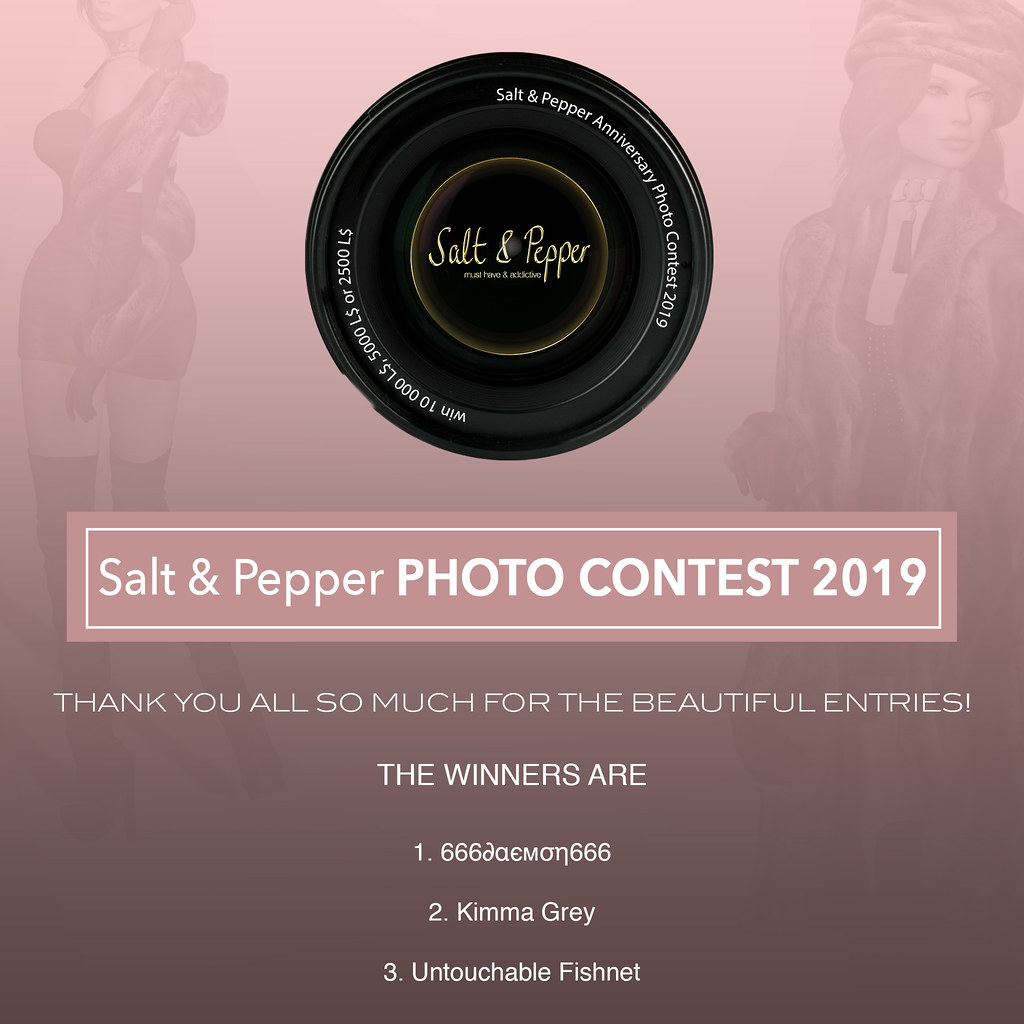The image features a computer banner for the "Salt and Pepper Anniversary Photo Contest 2019." Dominating the center is a black circular graphic with a smaller, centrally-located brown circle bearing the text "Salt and Pepper" in a stylized script. Encircling the black circle is further text indicating the contest's name and tantalizing reward amounts: "Win 10,000 L$, 5,000 L$, or 2,500 L$." The banner is set against a gradient pink background that transitions from light to almost black towards the bottom. Directly below the central graphic, a pink rectangular banner with a white border and white text proclaims "Salt and Pepper Photo Contest 2019." Following this, a white-font message expresses gratitude for the entries and announces the winners: "Thank you all so much for the beautiful entries. The winners are: 1. 666 Damon666, 2. Kimma Gray, 3. UntouchableFishnet." Framing this content, faint images of two sexily-dressed, stylized women—likely computer-generated or hand-drawn—are positioned in the background on the top left and right corners.